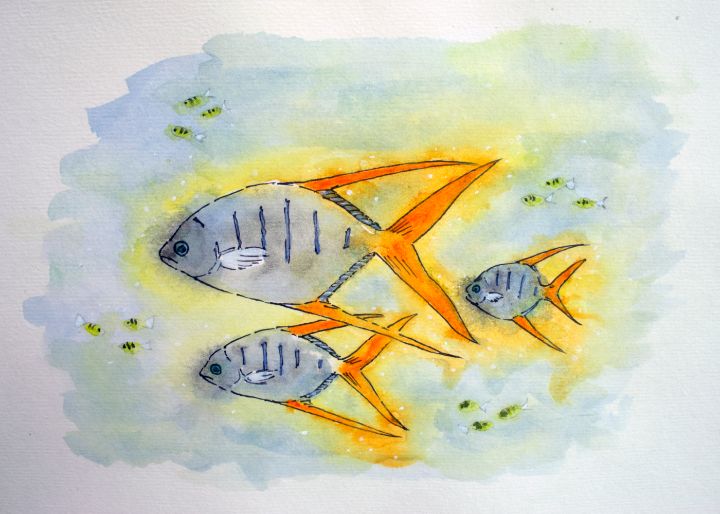This detailed watercolor painting, likely created on a white, slightly textured canvas, illustrates an underwater scene with three larger fish swimming gracefully in the center. The fish have elegant grayish-blue bodies with white wing-like fins around their gills. Their dorsal, ventral, and tail fins are long, slender, and painted in a bright orange hue. The largest fish is positioned towards the top left, with a slightly smaller fish beneath it and an even smaller one trailing behind. Surrounding these main fish are several smaller groupings of fish, four in total—distributed as follows: one group in front of the lead fish, one above, and two trailing behind the rearmost fish. These smaller fish are vibrantly yellow with black stripes and white tails, adding a lively contrast to the central scene. The center of the canvas also features subtle touches of pale blue, yellow, and orange, enhancing the sense of depth and movement within this captivating underwater tableau.